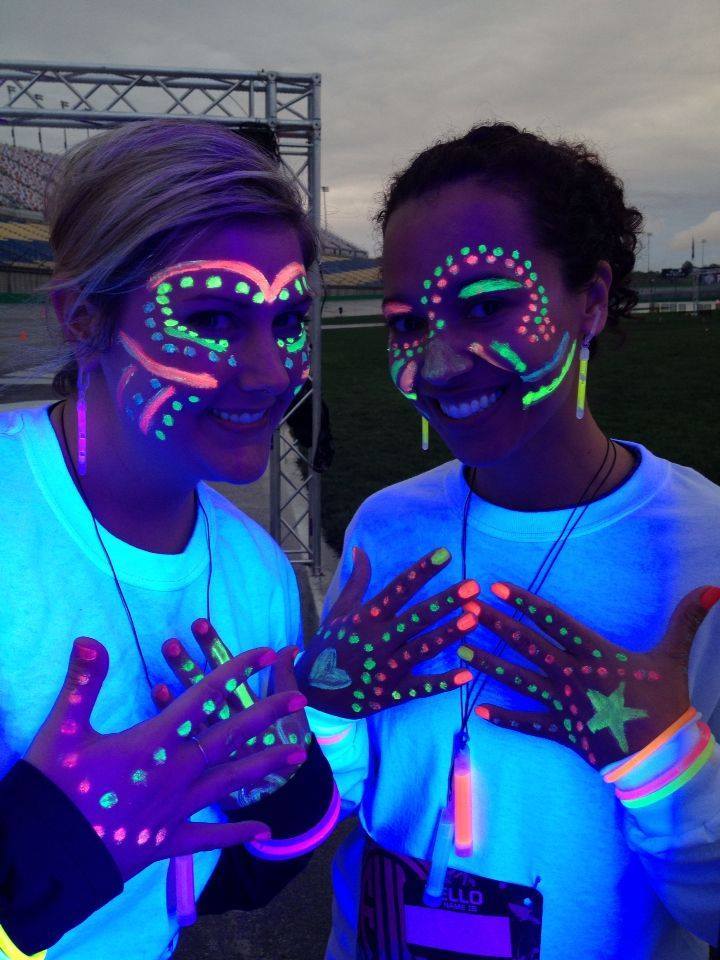In this photograph, two women are adorned with intricate black light paint, creating a vibrant, glowing effect under ultraviolet light. Both are dressed in white shirts that also glow under the black light, adding to the luminous scene. The women’s faces and hands are covered in patterns of fluorescent dots, lines, and curves. The woman on the left, with blonde hair, features orange eyebrows and a series of green and pink dots around her eyes, cheeks, and fingers. The woman on the right, with curly hair, showcases a similar motif of pink and green dots, particularly concentrated in a 'hump' shape on her face. Both have glow sticks serving as earrings and wear glowing necklaces—one in neon orange and the other in purple—complementing their overall glowing appearance. Additionally, the individual on the right sports several glowing bracelets and a distinctive light blue star painted on her left hand. The setting suggests an event like a rave or concert, enhancing the lively and energetic atmosphere captured in the image.